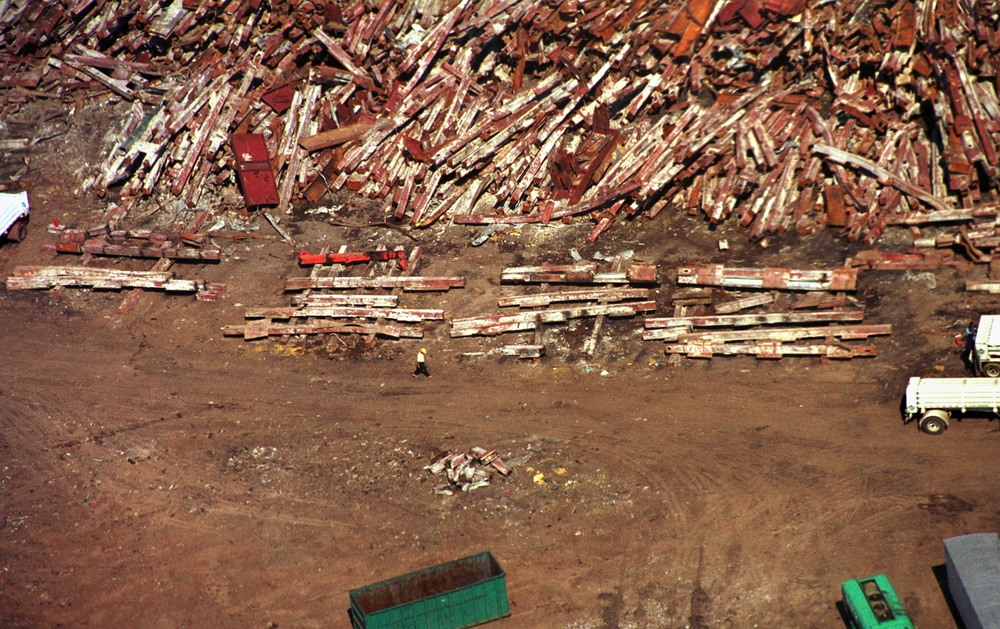This is a horizontally oriented, top-down aerial photograph of what appears to be a construction site or junkyard. The scene is dominated by a dirt ground, with a variety of debris and trash scattered throughout. At the very top, there are numerous rectangular pieces, possibly made of wood or tree branches, predominantly in different shades of red and white. Below this is a segment with similar material laid out in neat rows and columns. A figure can be seen walking along the edge of these materials. In the middle right section, a long white truck is driving away, creating a contrast against the dark brown dirt road. Toward the bottom center of the photograph, a green trash bin or dumpster is prominently visible. In the lower right corner, there's a green vehicle and the corner edge of a gray building. Overall, the photograph captures the chaotic yet structured nature of the site with various trucks, containers, and debris laid out across a dirt embankment.